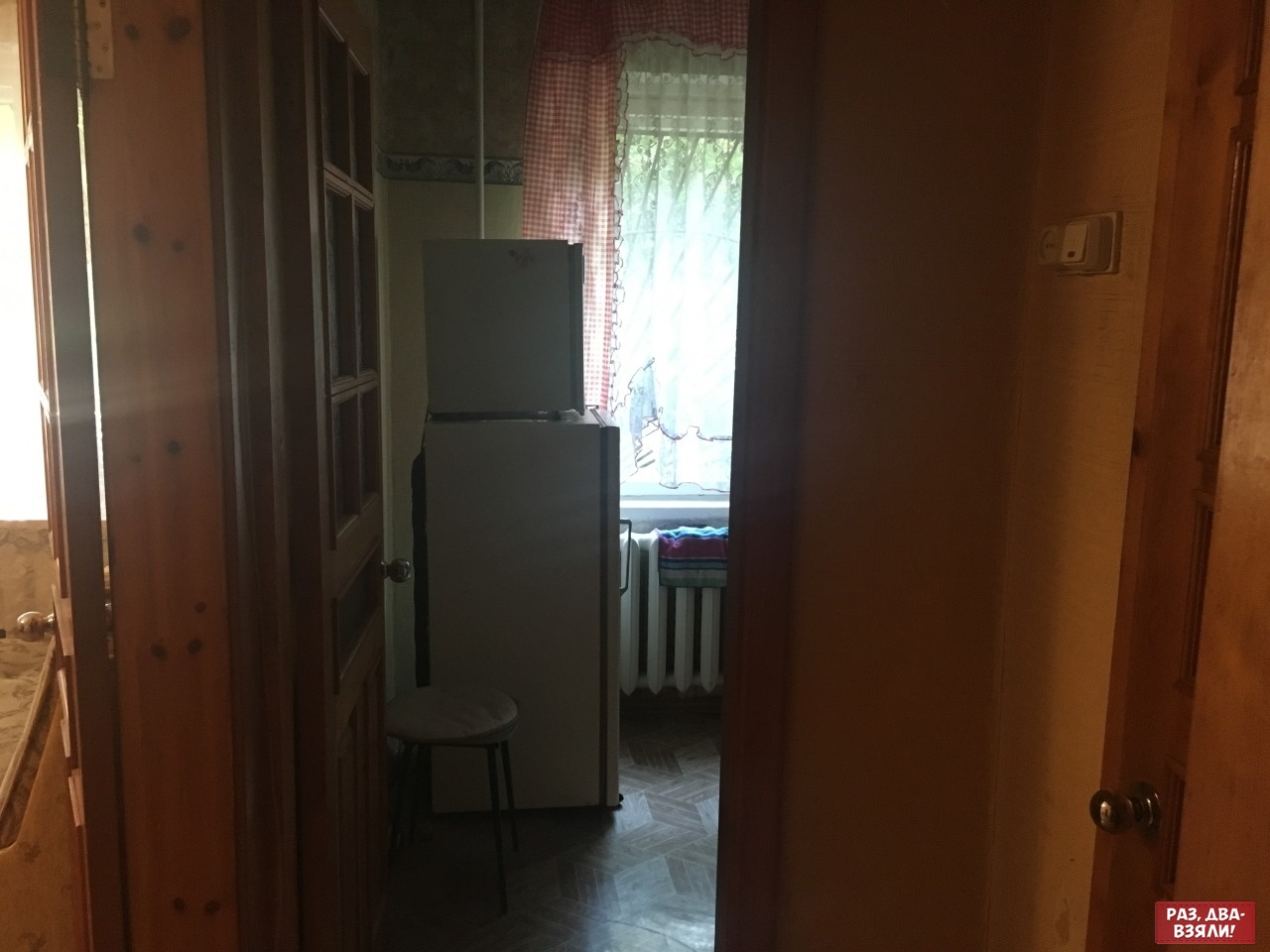The image depicts a view into a kitchen from a wooden hallway in a house. The foreground reveals wood paneling and trim, characteristic of the home's interior. On the left, there's an open wooden door with a gold handle, leading into another room, possibly revealing a mattress. To the right, a partially visible closed wooden door stands beside a beige, chipped wall that hosts a thermostat. In the center, an open wooden door with six glass panels leads into the kitchen. Inside the kitchen, a white round stool, possibly holding the door open, sits in front of a white refrigerator. On top of the refrigerator is a smaller white appliance, potentially a microwave or compact freezer. A vintage-style white radiator, draped with a blue and red towel, is installed below a window adorned with semi-translucent pink curtains with red and white plaid edges, which let in natural light and reveal a glimpse of green leaves outside. The kitchen walls are white with a floral trim around the top, and the floor appears to have a parquet design.